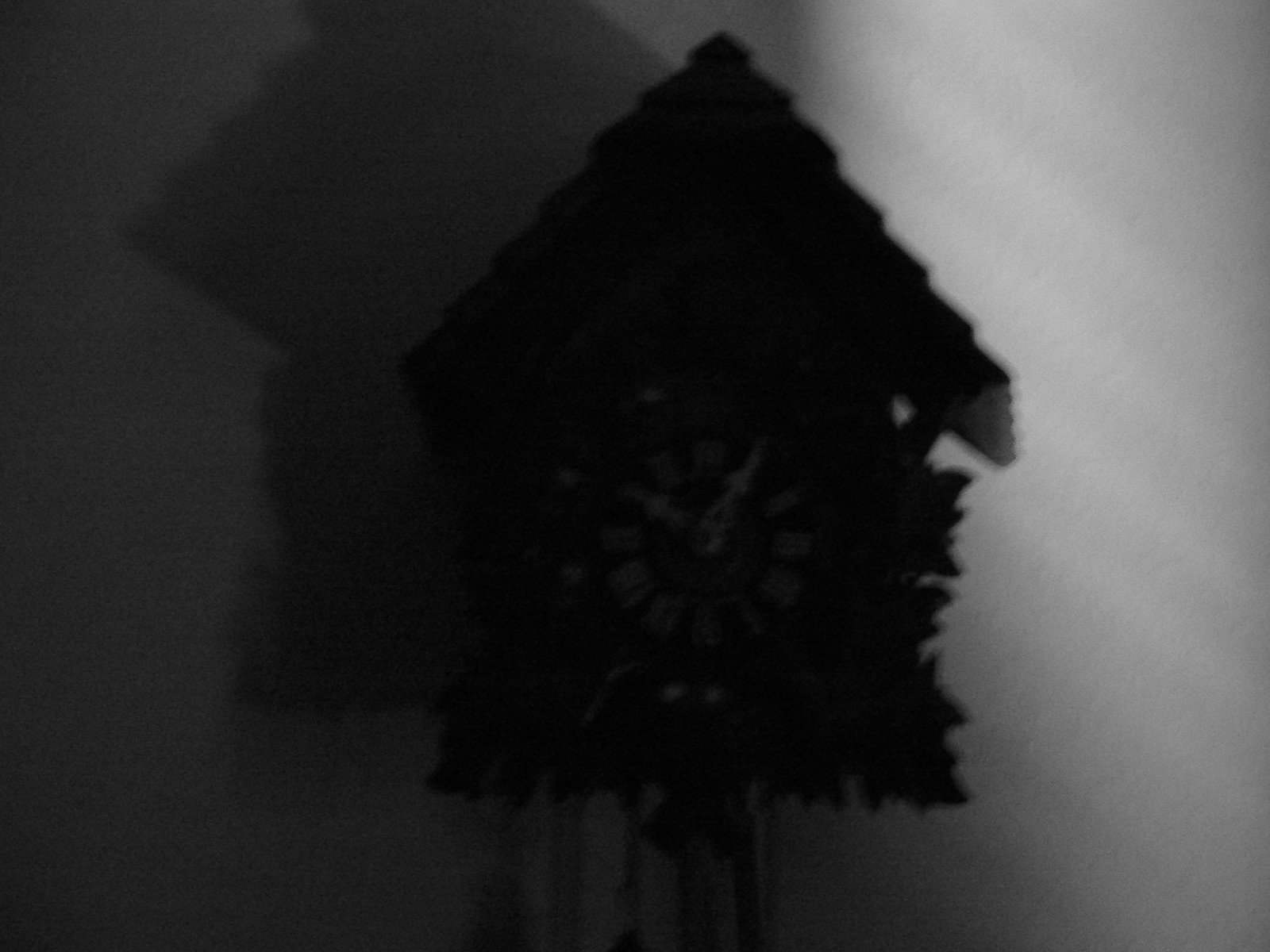This black and white image features a dark, grainy photograph of a cuckoo clock set against a white background, creating a strong contrast that defines the object’s silhouette. The left side of the image is significantly darker, making the shadow of the cuckoo clock, cast to the left, more prominent, while the right side is illuminated by a light source coming from the bottom right. The clock itself has a textured, possibly leaf-like, jagged edge along the sides, forming a distinct silhouette. It is A-framed with a peaked rooftop and intricate, natural wood grain details, giving it an organic appearance.

The face of the clock is black with striking white Roman numerals and hands, displaying a time around 10:05. Although the image suggests the clock might be dark brown, the low quality and lighting make it difficult to discern this precisely. Hanging from the clock are what appear to be chimes, though the photo’s darkness prevents the ends from being visible. The entire scene is shadowy, with the granular composition and subtle light gradients emphasizing the antique, almost eerie character of the cuckoo clock.